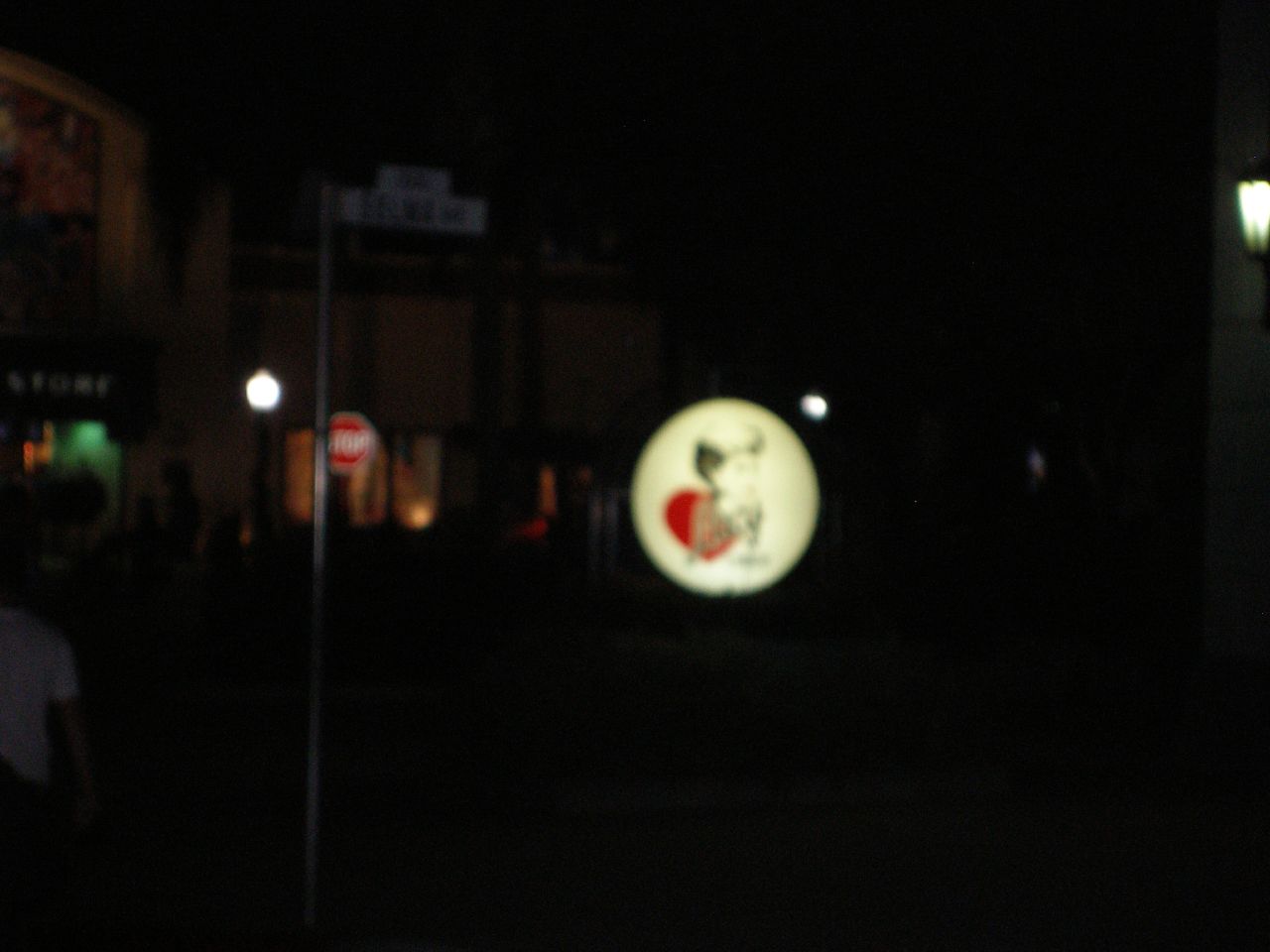A nighttime, first-person POV photograph captures a somewhat circular, white LED-lit sign, emblazoned with an indistinct graphic that appears to depict a baby fox with a heart-shaped tail. The sign and surrounding scene are slightly blurry and grainy, implying motion during capture or the use of a low-quality camera. The dark sky is punctuated only by a few lanterns, contributing to the ambient lighting. To the left of the photo, a building with illuminated windows can be seen, indicating that it is open and likely the establishment associated with the sign. Outside, a black silhouette of a person is visible, seated near the doorway, which is partially obscured by a black retractable cover displaying an incomplete, unreadable business name. In the lower left corner, the partial figure of a person in a blue shirt is seen walking out of frame towards the lit building, adding a dynamic element to the tranquil, night-time scene.